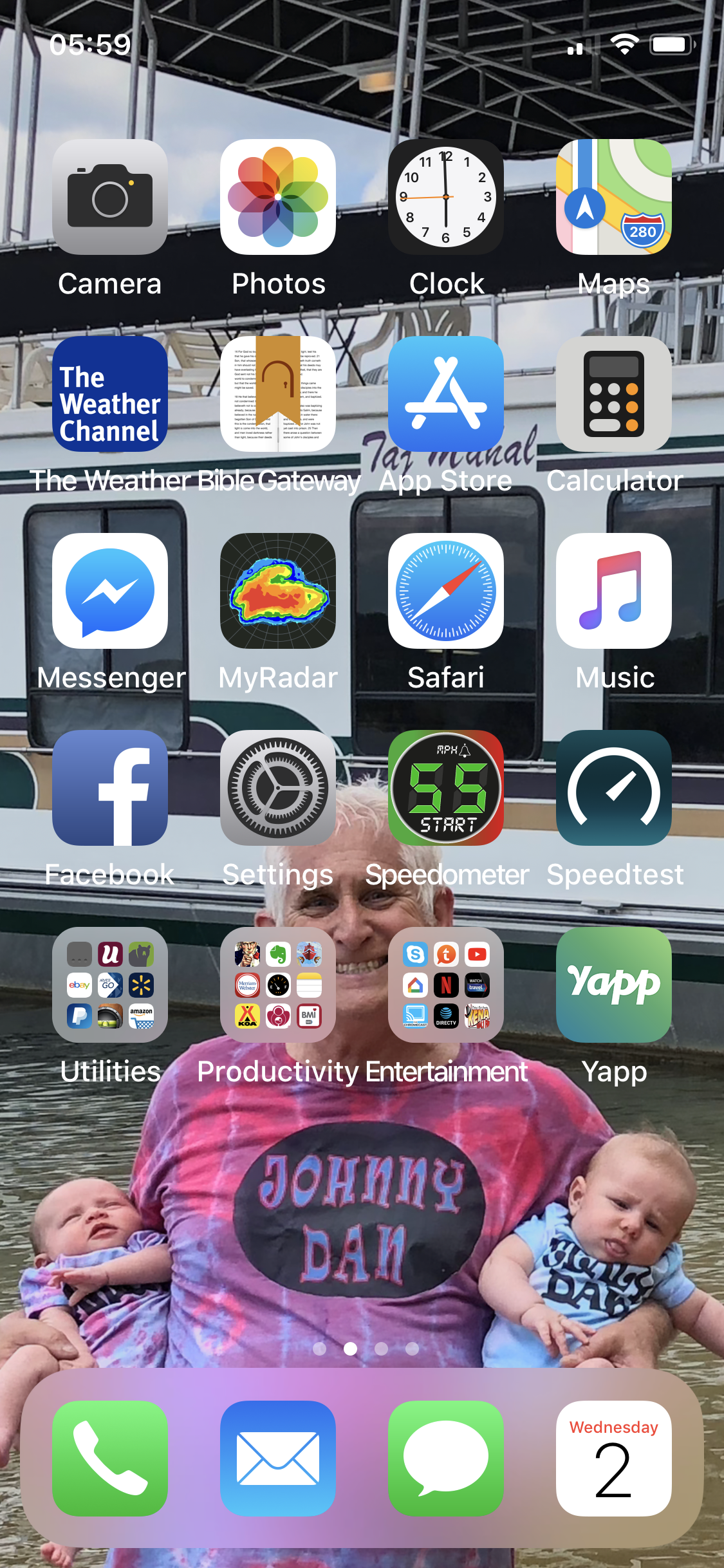In this image, we see an iPhone screen with various icons prominently displayed, partially obstructing the background. Despite the icons, the focus is on a heartwarming scene featuring an elderly man, presumably a grandfather, holding two young babies. The grandfather wears a vibrant t-shirt with a black circular emblem that features the text "Johnny Dan" written in blue lettering with a red outline. His t-shirt is a colorful mix of patterns, adding more vividness to the scene.

One of the babies, positioned on the right, is dressed in a bright blue t-shirt, while the other baby, on the left, wears a tie-dye colored shirt with shades of pink, purple, and blue, resembling the grandfather's shirt. Behind them, there appears to be a train in a station, though the train's name is partially obscured by the screen’s icons, making it difficult to read. This lively and touching scene captures a moment of familial joy against the backdrop of a busy train station.